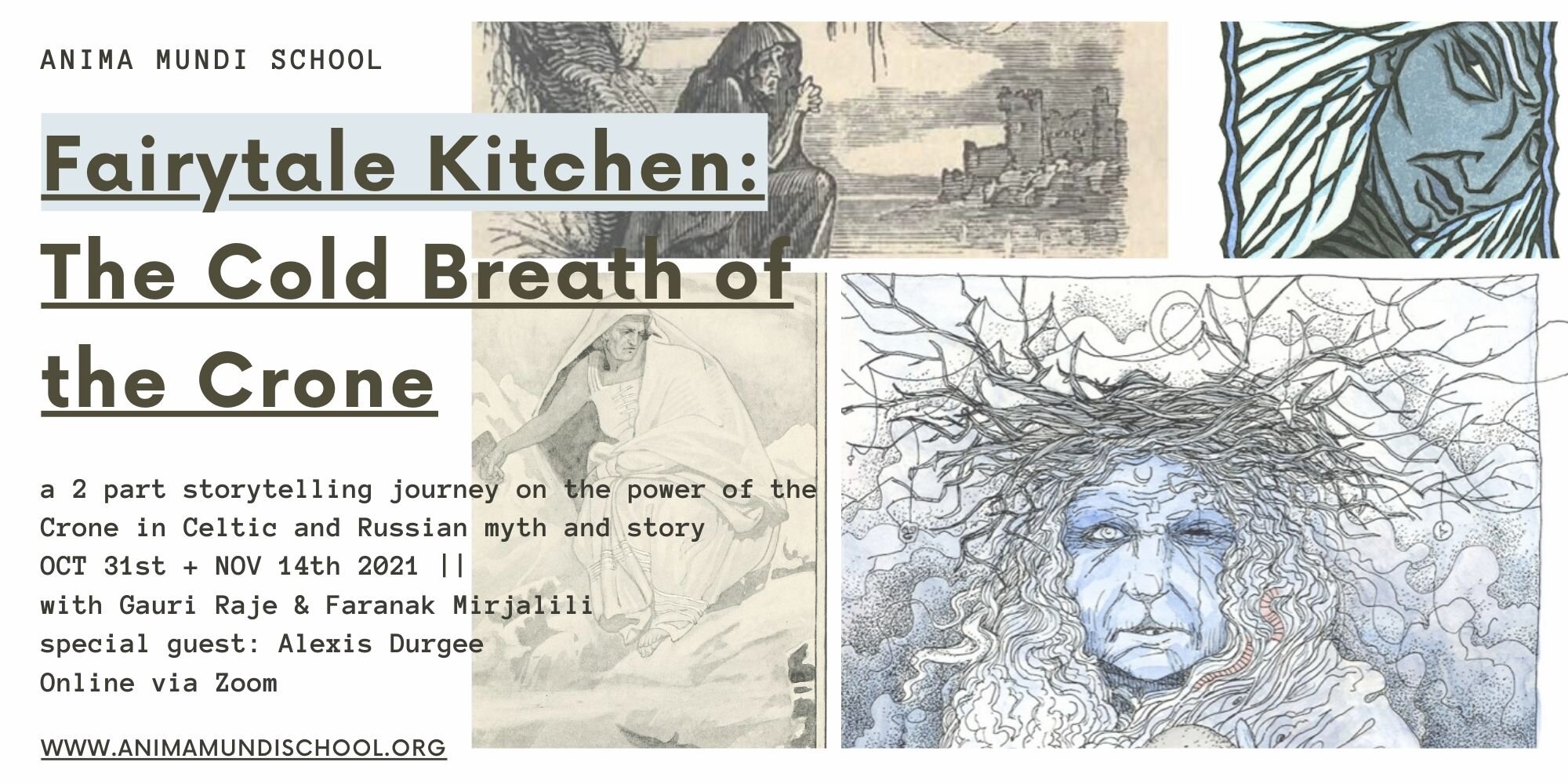This horizontally vertical print advertisement features a simple color palette of two to three colors with a clear, white background on the left side, occupying around 25% of the space. The top left corner showcases the text "Anima Mundi School" followed by the headline "Fairytale Kitchen: The Cold Breath of the Crone." Underneath, the text states, "A two-part storytelling journey on the power of the Crone in Celtic and Russian myth and story, October 31st through November 14th, 2021, with Gauri Raje and Faranak Mirjalili, also guest Alexis Dergy," and the event is noted to be online via Zoom. A URL at the bottom left reads www.animamundischool.org.

On the right side, four hand-drawn images depict crones, which are likely the focus of the storytelling event. The uppermost drawing is of an elderly figure with twigs for hair, a wrinkled face, and an eye that appears closed or missing. Below that is an ominous face with long white hair and piercing, malevolent eyes. To the left of this figure is a depiction of a witch in a cape beside a castle. The bottom drawing features a lighter sketch of a person in a white robe with a hood. The two drawings on the right are tinted with blue-colored pencil, adding to the eerie and mystical theme. Together, these elements combine to evoke the crone's powerful and mysterious presence in folklore and mythology.